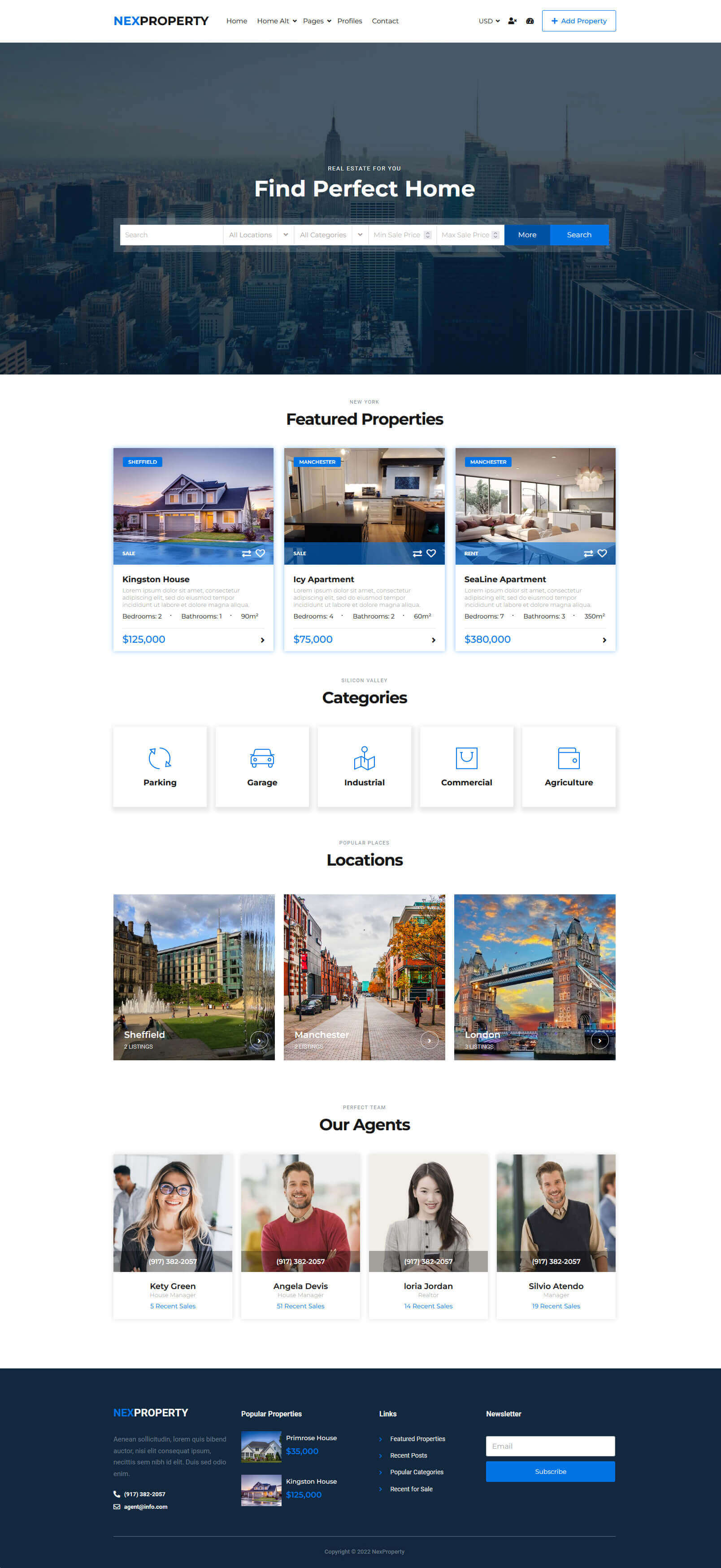In this screenshot from the Next Property website, the upper left-hand corner features several small, unreadable buttons. A search bar with the text "Find Perfect Home" rests atop a cityscape image. Below, a section titled "Featured Properties" displays three photos: the exterior of a house, a kitchen, and a living room. Further down, categories like Pricing, Garage, Industrial, Conventional, and Agriculture are listed. The "Location" section follows, showing Sheffield, a pixelated middle location, and London, each illustrated with respective images. Finally, the bottom section, "Our Agents," presents photos of four team members.